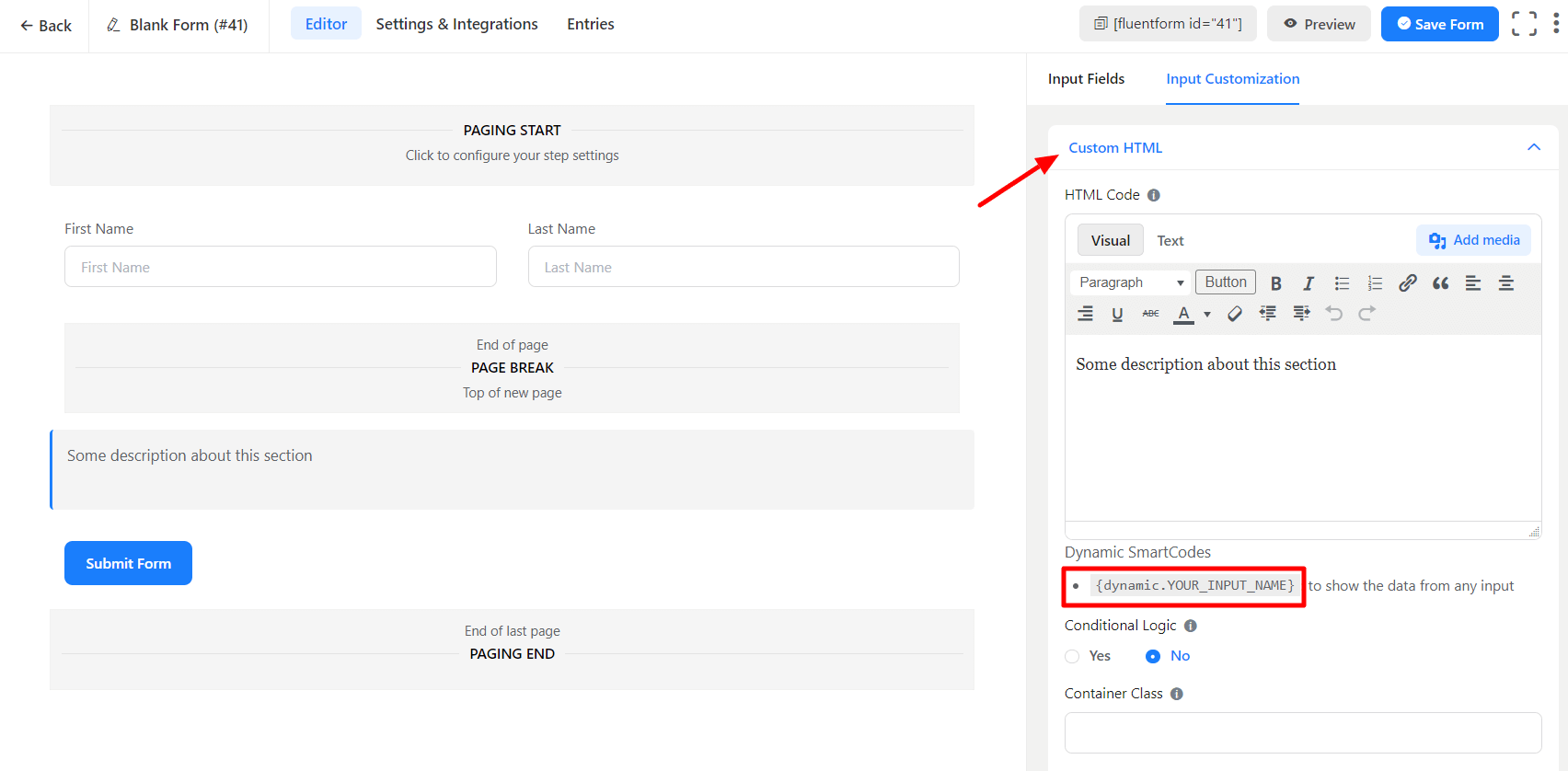The image captures the screen of a computer showcasing a user interface with a split layout. 

On the left, a wider section prominently displays "Blank Form Number 41" at the top, with an editor menu featuring tabs: Settings, Integrations, and Entries. Below this menu, the interface invites configuration with a prompt that reads "Click to configure your step settings." The main form begins here, requesting the user's first name and last name with text input bars provided for each. Following this input field, there is a gray bar labeled "End of Page Page Break," indicating a transition to the next page. A description follows, which leads to a "Submit Form" button. The section concludes with the text "End of Last Page Paging End."

On the right side, a narrower area mimics the appearance of a mobile device interface. The top features controls such as Preview, Save Form, Input Fields, Input Customization, and a Custom HTML option. Highlighted by a red rectangle, "Dynamic Smart Codes" are prominently displayed, suggesting a focus on custom coding or script integration within this form view. This dual-pane setup allows users to configure and preview the form simultaneously on a computer and mobile interface, ensuring responsive design and functionality across devices.